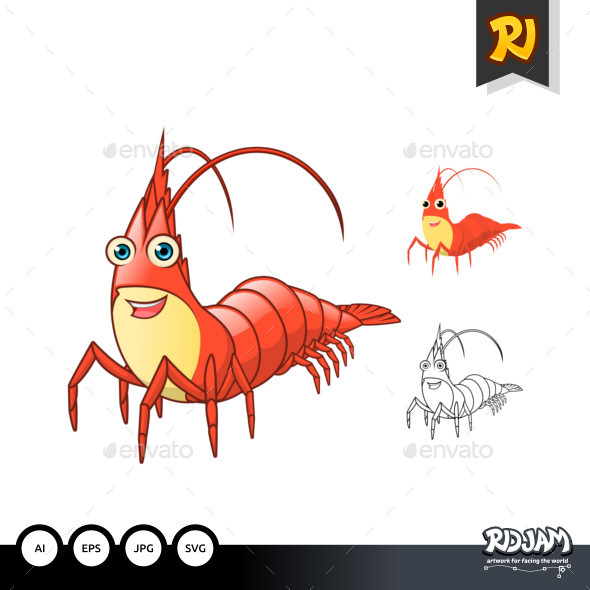This image features a trio of cartoon-style crustaceans set against a white background with a diamond pattern, with the word "ENVATO" interspersed between the diamond points. On the left side of the image is a large, red crab with a smiling, human-like mouth and blue eyes. The crab's body is red with a yellow underbody and around its mouth. It has numerous thin legs, two long red antennas, and the shape of a peak at the top of its head. To the right of this crab are two additional illustrations: a smaller crab that shares the same red body and yellow chest but has black eyes, and below it, a black-and-white outline of the same crab. In the upper right corner of the image, there's a bookmark icon labeled "RI," and at the bottom, a black banner with four white buttons labeled "AI," "EPS," "JPG," and "SVG," with "RDJAN" written in white on the far right of the banner.